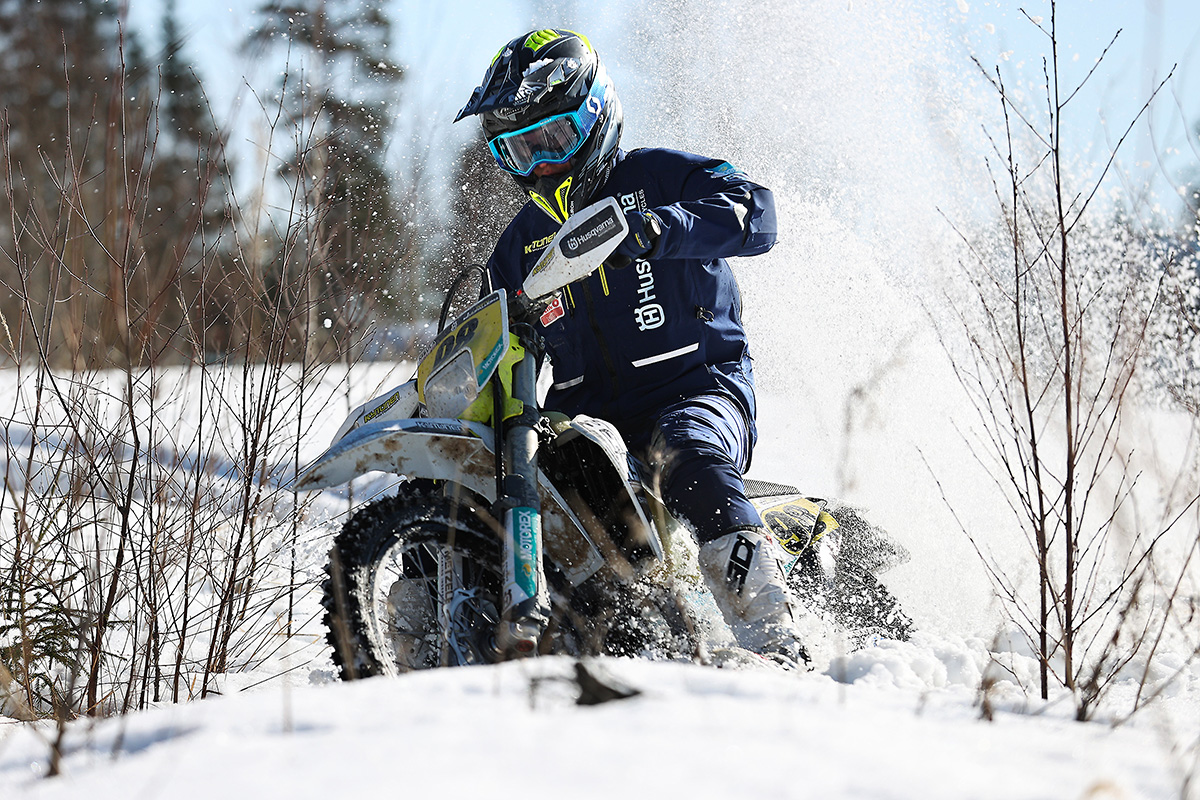This daytime outdoor photograph captures a man navigating a snowy landscape on a dirt bike. He is captured mid-turn, with his front wheel angled to the right, creating a spray of snow behind him that arcs like a wave. The man is clothed in protective winter gear, including a thick dark blue jacket, matching dark blue pants, and white boots. His head is protected by a black and yellow helmet, and he wears blue-tinted ski goggles that obscure all but his nose and the high collar of his jacket. The dirt bike itself is a mix of white, blue, and yellow, with a visible number on its front. Surrounding him is a snowy field, dotted with small saplings poking through the snow. The background shows more snow-covered fields with faint tire marks, possibly indicating a makeshift roadway, and trees standing at a distance against a bright, clear sky. The scene exudes the crisp, cold atmosphere of winter, and the man appears fully concentrated on maneuvering his bike in this challenging environment.